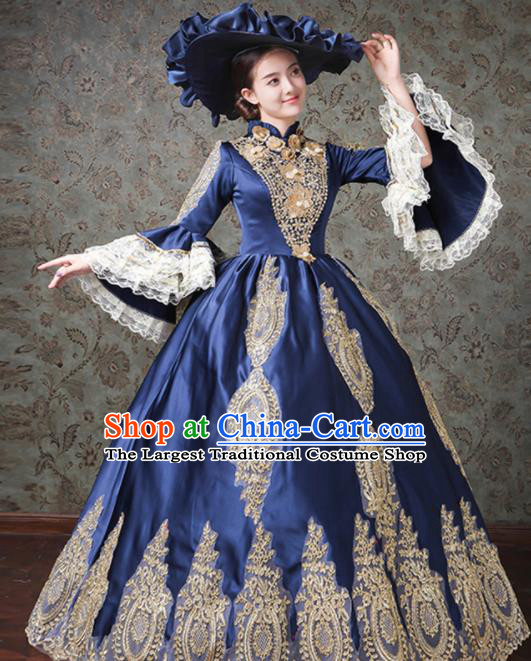The photograph captures an elegant scene featuring a young Asian model, likely in her mid-20s, with fair skin and brown hair styled into a bun. She is adorned in an elaborate, navy blue satin gown reminiscent of early 19th-century British royal fashion. The dress features intricate gold lace detailing around the bodice and under the skirt. The sleeves are designed with bell-shaped white frills at the ends, emphasizing the vintage aesthetic. Complementing her attire is a large, ornate hat, resembling those worn at Kentucky Derby events, complete with blue ruffles. Standing gracefully, the model's slender frame is accentuated by the voluminous, bell-shaped lower portion of the gown.

The background sets a sophisticated tone with dark gray and greenish wallpaper embellished with brown floral patterns, a wooden baseboard, and brown hardwood flooring. The entire image exudes a historical ambiance, enhanced by the ornate decor.

Superimposed text spans the center of the gown: 
- "Shop" in red letters with white outlines 
- "at" in green letters with white outlines 
- "China-Cart.com" in blue letters with white outlines, underlined 
- Below is the tag line in black letters with white outlines: "The Largest Traditional Chinese Costumes Shop."

This detailed composition offers a striking visual of classic elegance fused with a touch of cultural heritage marketing.